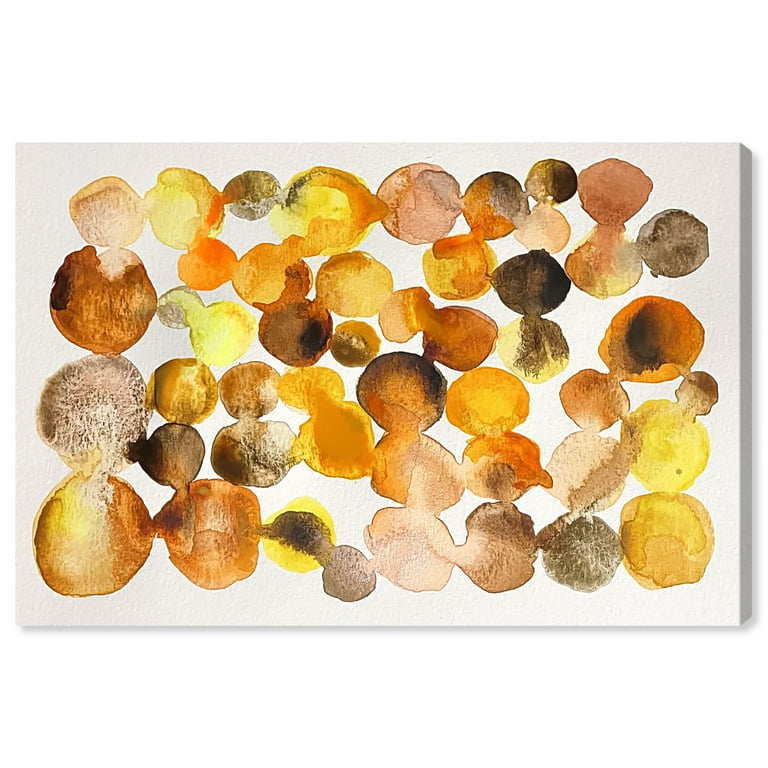The image depicts an abstract painting on a light gray or off-white canvas, which appears to be mounted on a wooden frame. The painting is filled with pairs of irregular, ring-shaped forms that resemble dried slices of vegetables in hues of brown, yellow, orange, dark orange, beige, tan, and dark brown, with hints of light brown and black. These shapes are arranged predominantly in vertical orientations although some are angled differently. The depiction of these objects creates a visually rich, warm-colored ensemble that nearly forms a dumbbell shape in some pairs, while others connect in a seemingly random pattern. This intricate, hand-painted artwork suggests the texture of faceted surfaces, and the photograph emphasizes the vividness and randomness of the connected and disconnected colored circles, drawing attention entirely to the painting itself, either hanging on a wall or viewed from above.